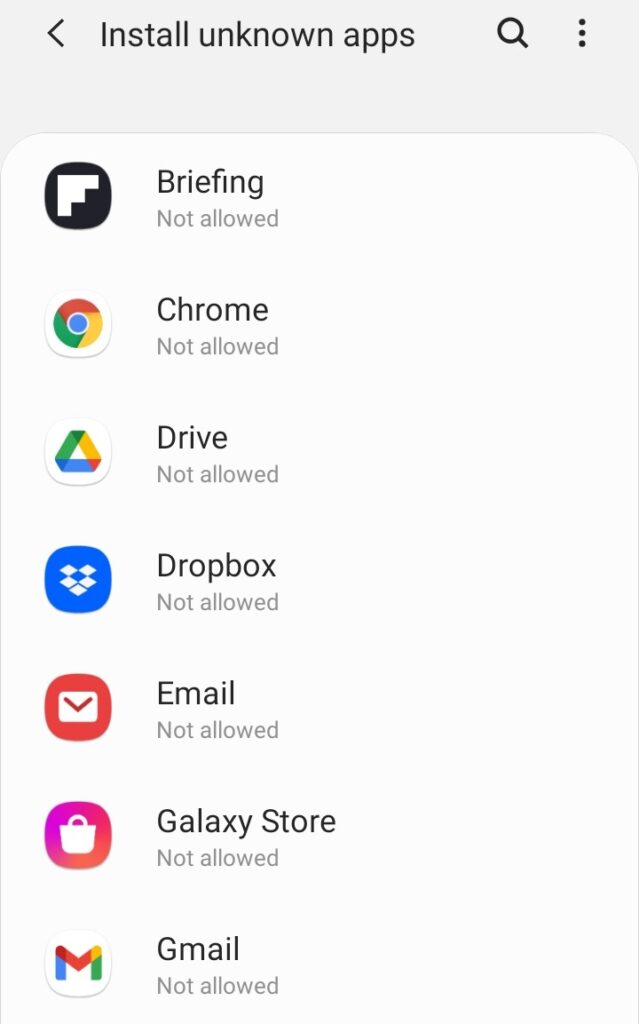The image displays a smartphone screen showing a list of apps that are restricted from being installed from unknown sources. The apps listed include Briefing, Chrome, Drive, Dropbox, Email, Galaxy Store, and Gmail, all marked as not allowed. The individual who set these restrictions appears to be taking extra precautions to protect their device, which is likely an Android phone, as indicated by the mention of the Galaxy Store. This vigilant approach demonstrates a commendable effort to maintain cybersecurity and manage app permissions effectively.